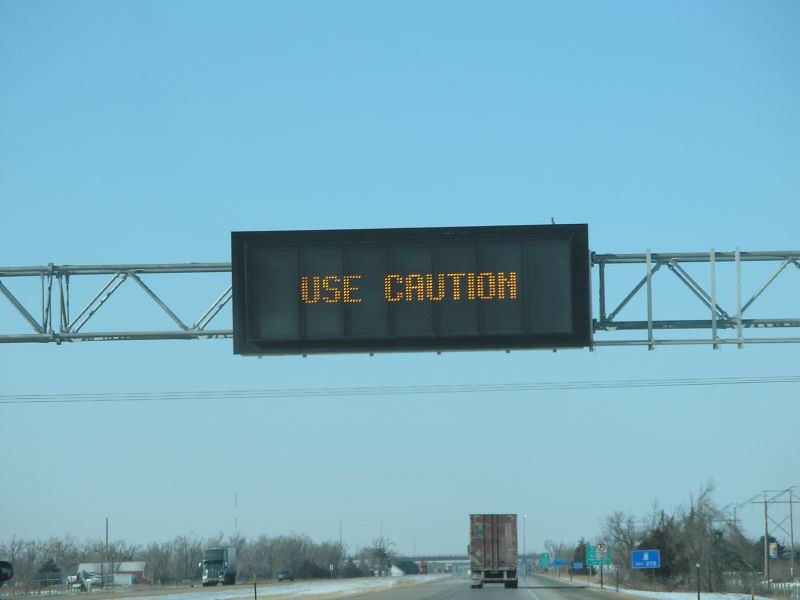In this detailed photograph taken on an interstate highway under a clear blue sky, a scene unfolds with various elements drawing the eye. The viewer’s perspective is from behind a semi-truck towing a faded red trailer, traveling along a snow-patched road. Snow is intermittently present on the road and gathered along the edges. On the right-hand side of the frame, the semi-truck looms prominently while another truck approaches from the opposite direction on the left-hand side.

The roadsides are flanked with numerous signs, including a blue rectangular sign with a gas pump icon and a white square sign featuring a red circle with a diagonal line over a black “P,” indicating no parking. Additionally, there are several green signs, though the exact details are difficult to discern. The backdrop reveals trees mainly devoid of leaves, with the exception of a single tree still bearing some foliage.

Prominent in the middle of the image, a metal pole supports an overhead black sign with bold, neon orange letters, emphatically instructing travelers to “USE CAUTION.” In the distant background on the left, a house or barn subtly peeks into view. Finally, ahead on the highway, an overpass bridge looms, marking yet another feature of this richly detailed roadside scene.